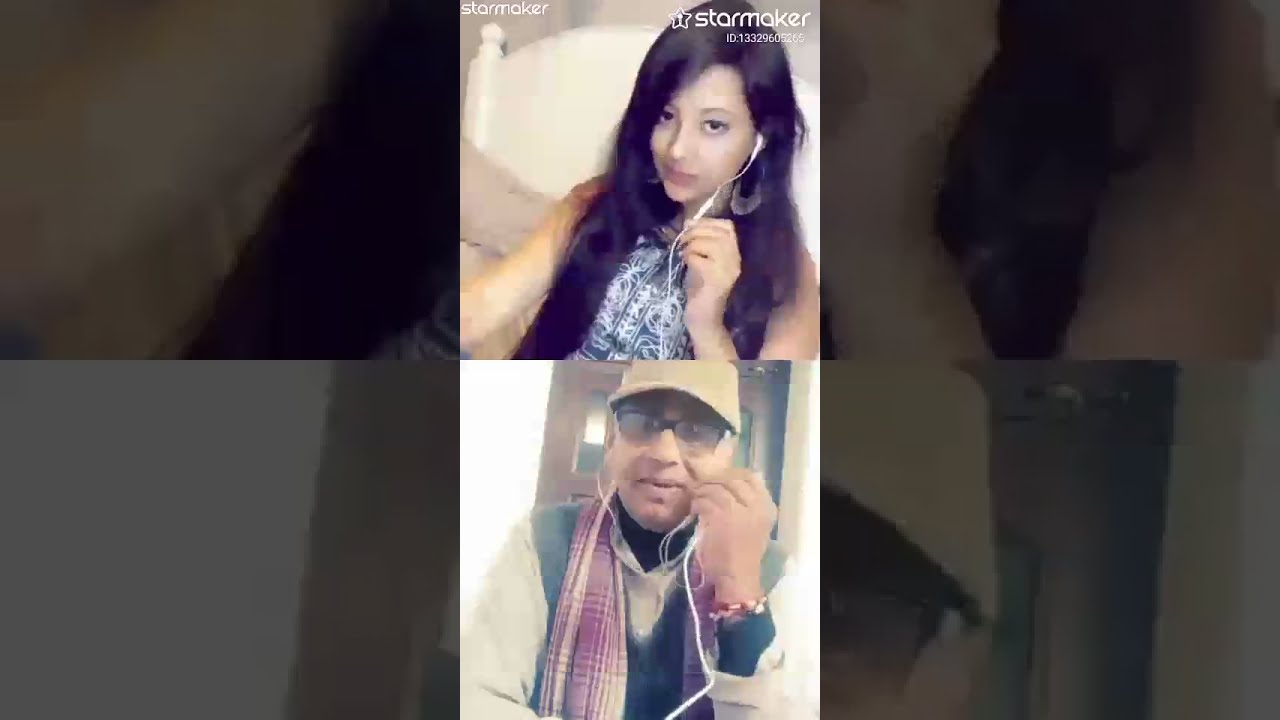The image is a color photograph comprising two separate photographs stacked vertically. Both images show a young woman and a man engaging in an online conversation via an app interface. The top photograph features a young woman with brown skin and long dark hair, looking up at the camera. She is wearing white earbuds with a cord that she is holding in her left hand. She is dressed in a black and white patterned top, and her background includes a white bed frame. The interface displays the words "Star Maker" in white text in the upper left corner, and a star logo with "Star Maker" and an ID number in the upper right corner. 

Below her, in the second photograph, is a man with brown skin wearing a tan-colored ball cap, thick black-rimmed glasses, and a red and white plaid scarf over a green vest and white shirt. He is also wearing white earbuds and holds the cord in his hand, seemingly speaking into it. He gazes directly into the camera. The background features a close-up of the interior of his home. The presentation style is distinctive, with the central images sharply focused while the peripheral areas display a faded, out-of-focus, black-and-white version of the same photographs, adding depth to the visual structure.